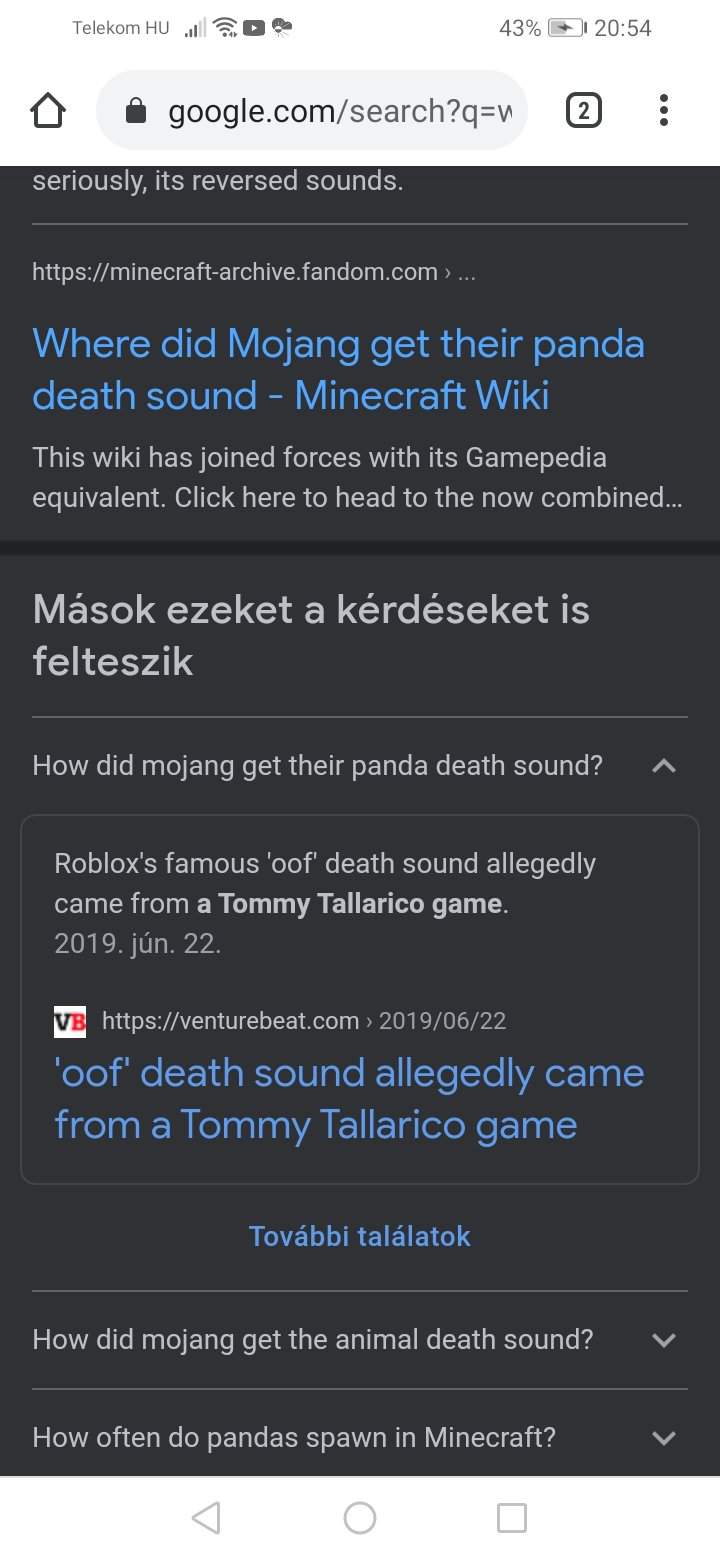In the upper part of the image, some small, unreadable text sits at the top. Beneath this, a series of bars increase in height from left to right; three bars are black while two are gray. A Wi-Fi symbol is present next to a small, black, right-pointing rectangle that resembles an arrow. Following this, there are two black circles accompanied by a small dot below them, and to the right, "43%" is displayed next to a partially filled battery icon. The time reads "20:54."

Below these elements, an upward-pointing arrow is visible. A light gray rectangle bulges at the ends, signifying it might be clickable or interactive. Inside this rectangle is a lock icon, followed by the URL "google.com/search?q=" with the input "mW." A black-outlined square with the number "2" inside and three vertically stacked black dots appear next.

Further down, a black rectangle contains the text "Seriously, it's reverse sounds." Directly below this is a white line, followed by a hyperlink in blue text: "Where did Mojang get their panda death sound - Minecrave Wiki". This text explains the wiki’s merger with the Gamepedia equivalent and includes a clickable link to access the combined site. 

Below this, foreign text appears with characters such as "MÁ-SOKÉZÉKET," "KÉ-RDÉ-SÉKET," and "FELTÉS-ZIK." Another separator line is displayed beneath this section, reading "How did Mojang get their panda death sound?" followed by another upward-pointing arrow.

The next section details "Roblox's famous oof death sound allegedly came from a Tommy Tallarico game," dated June 22, 2019. A white square with the letters 'V' in black and 'B' in red accompanies a similar hyperlink: "Oof death sound allegedly came from a Tommy Tallarico game."

Following this, another string of foreign text is visible with characters like "TÓVA-BBITÁ-LA-BÁTOK." Below this, it reads "How did Mojang get the animal death sound?" with a downward-pointing arrow.

Finally, the image poses the question, "How often do pandas spawn in Minecraft?" with another downward-pointing arrow. Iconic gray-outlined shapes of a triangle pointing left, a circle, and a square complete the lower part of the image.